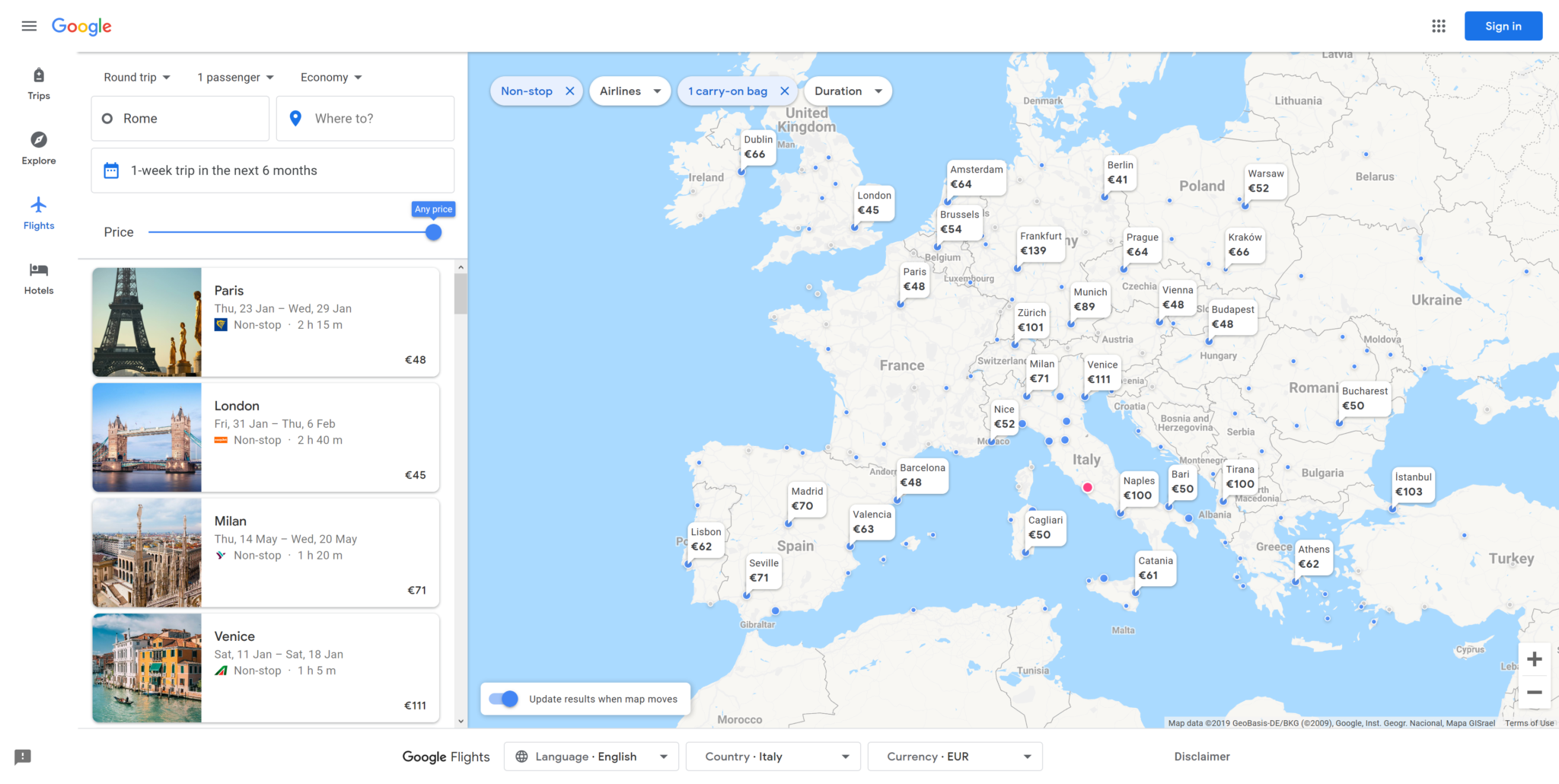The image is a detailed screenshot from Google Flights, showing an individual planning a one-week trip to Rome within the next six months. The interface highlights the search for flights, particularly displaying “Flights” in blue at the upper navigation bar. The word “Google” appears prominently in the upper right-hand corner, and at the bottom of the screen, the words “Trips,” “Explore flights and hotels” are visible, with “Flights” highlighted in blue. 

The search results emphasize non-stop flights to various European destinations, with prices ranging from $48 for Paris to $111 for Venice. Icons represent these cities with landmarks such as the Eiffel Tower for Paris, the London Bridge for London, notable statues for Milan, and a gondola scene for Venice. On the right side of the image, there's a map highlighting different European destinations including cities like Paris, Barcelona, Madrid, Italy, and Romania. 

At the top of the search results, there are filters for “Non-stop,” “Airlines,” “One carry-on bag,” and “Duration,” with “Non-stop” and “One carry-on bag” options highlighted in blue. The map, primarily blue and white, shows water bodies in blue and landmasses in white, clearly demarcating the European countries. In the bottom left corner, the option to “Update results for map moves” is highlighted.

Additionally, the map is dated from 2019, as indicated by a small note at the bottom, suggesting the data used is slightly outdated but still relevant for planning.